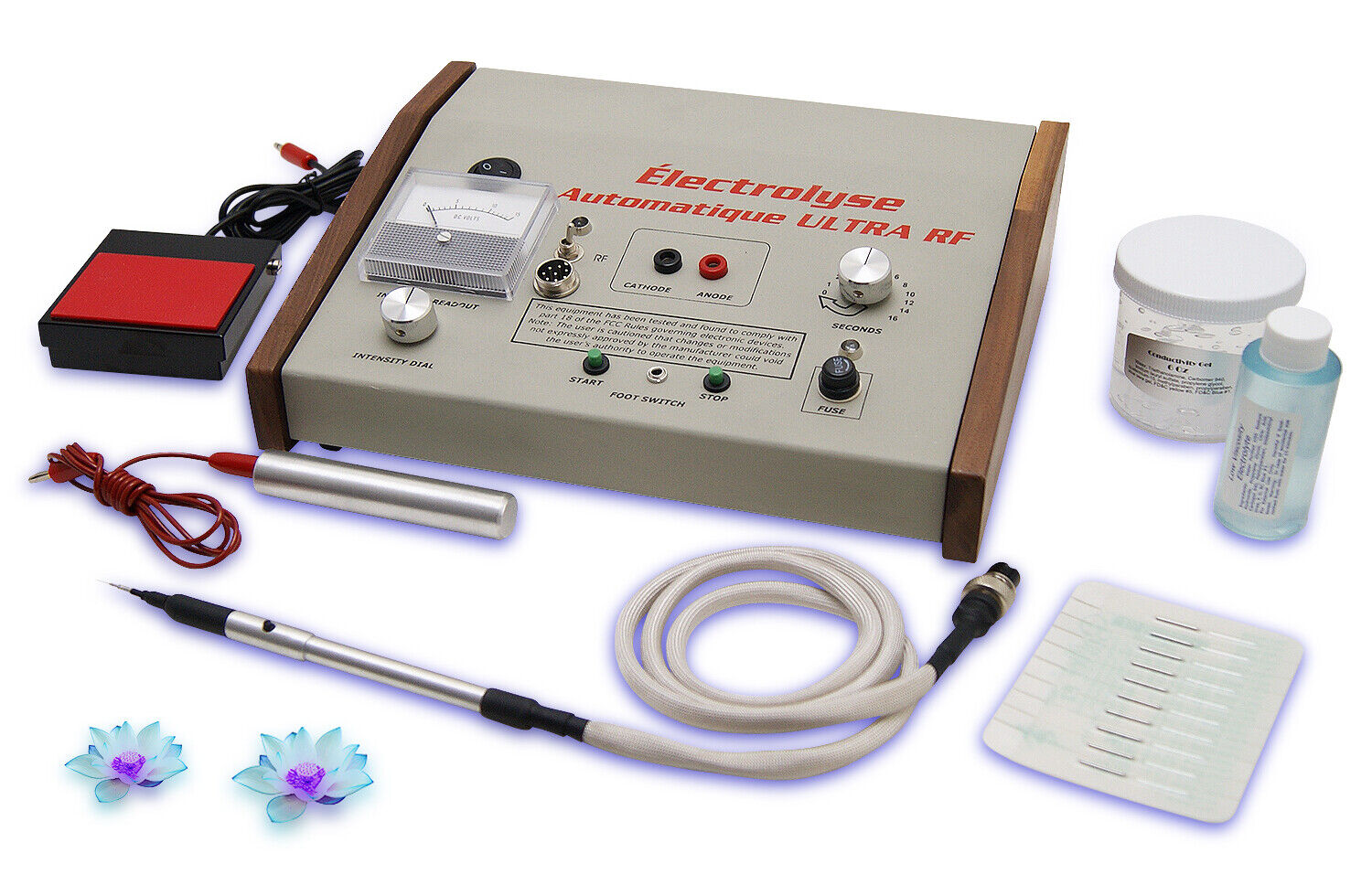The image is a detailed photograph of what appears to be a vintage medical electrolysis device, likely from the 1960s or 70s, labeled in French as "Electrolyse Automatique Ultra RF." The main machine, which has wooden edges on the left and right, features various controls including a central meter, a red plug, a black plug, two green buttons for start and stop, several dials including a pulse dial, and a root switch. Connected to the device are several accessories: a black rectangular pad, a silver tubular wand with a red cord, and a needle-like device, all of which plug into the main unit. To the right of the machine, there are two containers of gel, one being a jar and the other a bottle, with one containing clear liquid and the other a clearish-blue fluid. A pack of 10-12 replacement needle pins is situated next to the machine. The bottom left corner of the photograph features decorative artificial flowers, one being turquoise and the other purple, with purple gem centers.